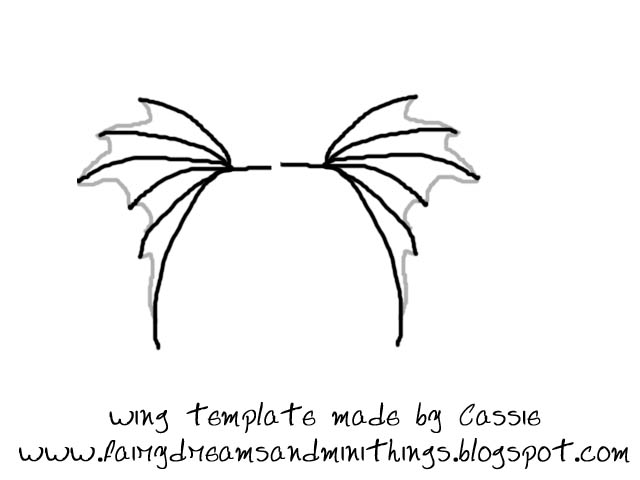The image features a detailed, black and gray drawing of symmetrical wings resembling either bat wings or angel wings. Each wing starts small at the top and gradually increases in size towards the bottom, with the last and longest wing extending prominently. The branches or bones of the wings are done in solid black, interspersed with white space between individual segments, suggesting a leathery texture rather than feathers. These wings are designed to attach at a crossbar behind a person’s back, indicated by a space for a body or head in the center. The entire image, which has a distinct silhouette or outline quality, gives an impression of either digitized artwork or a charcoal drawing set against a stark white background. At the bottom of the image, the text "wing template made by Cassie" directs viewers to the website www.fairydreamsandmanythings.blogspot.com, indicating the template is created by Cassie and possibly offered for sale or free on her blog.